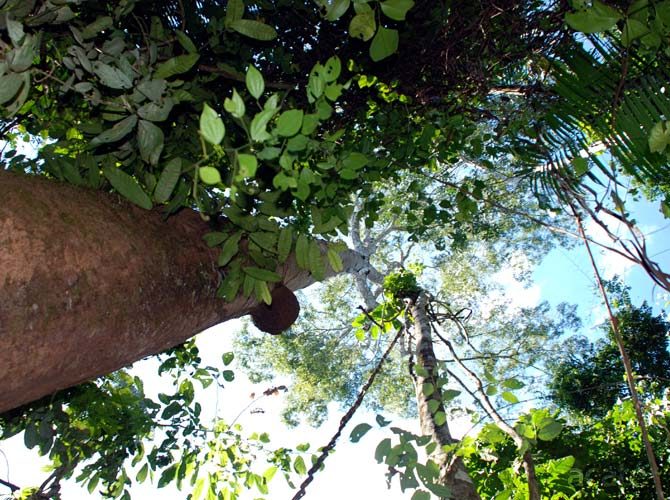This captivating horizontal photograph captures a unique perspective from the ground looking straight up into a serene blue sky dotted with white clouds. It vividly portrays a tranquil outdoor scene. Dominating the left side of the image is the brown trunk of an exceptionally tall tree, stretching up about 30 to 40 feet. The branches of this tree extend high into the air, framed by a plethora of leaves and shrubs that encircle the photograph's edges—top, sides, and bottom. Various types of greenery fill the upper area of the picture, including vines and fern-like leaves. The vantage point, as if the photographer is lying next to the tree with the trunk to their left, emphasizes the height and majesty of the tree and the surrounding foliage. The overall effect is an immersive upward view into nature's canopy, creating a sense of endless expanse and peaceful continuity.